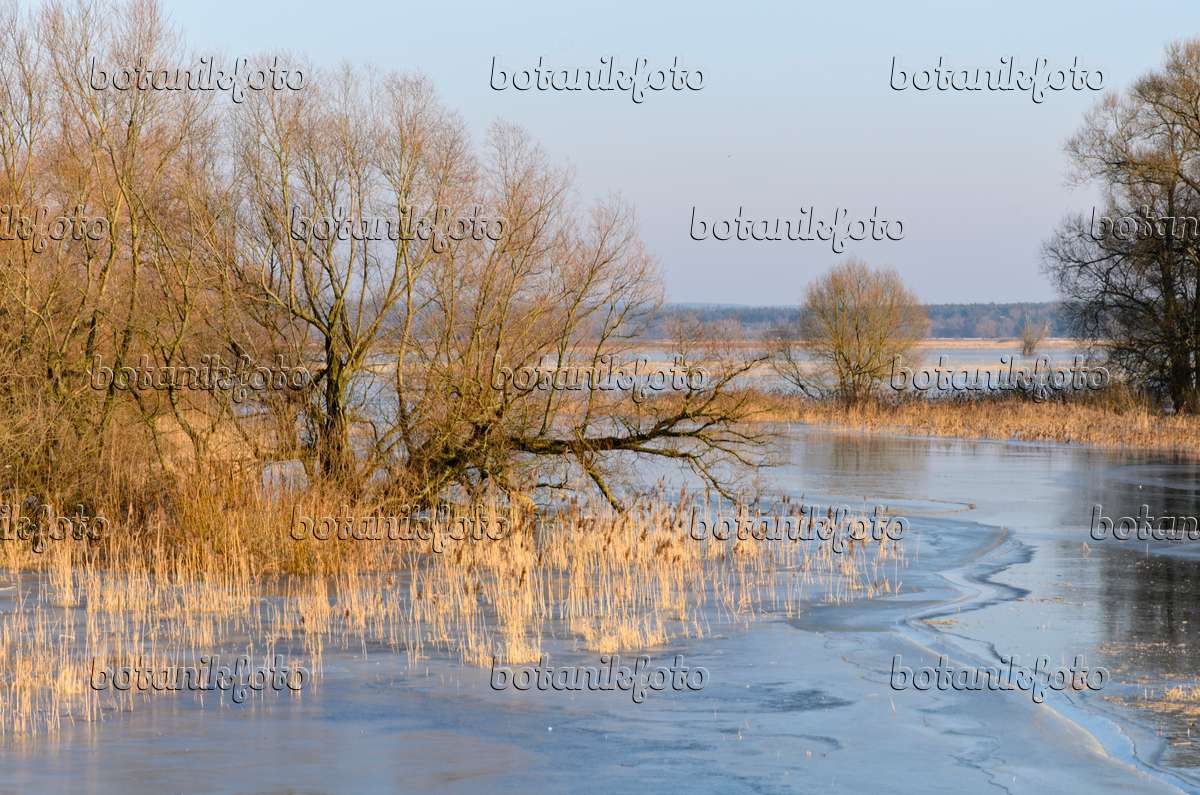The image captures a serene winter landscape centered on a lake, which appears to merge into a marshland. The water is dark blue and shallow, almost overflowing to the edges where barren trees and brush stand partially submerged. Among the yellow, wheat-like grass growing around the base of the trees, the frozen water subtly reflects the blues and whites of the sky and clouds. In the distance, the lake transitions into a marshy area dotted with small islands of dry grass and leafless shrubs, emphasizing the winter season. Transparent text saying "Botanic Photo" is scattered across the image from the left side to the bottom and upward to the right, serving as a watermark.